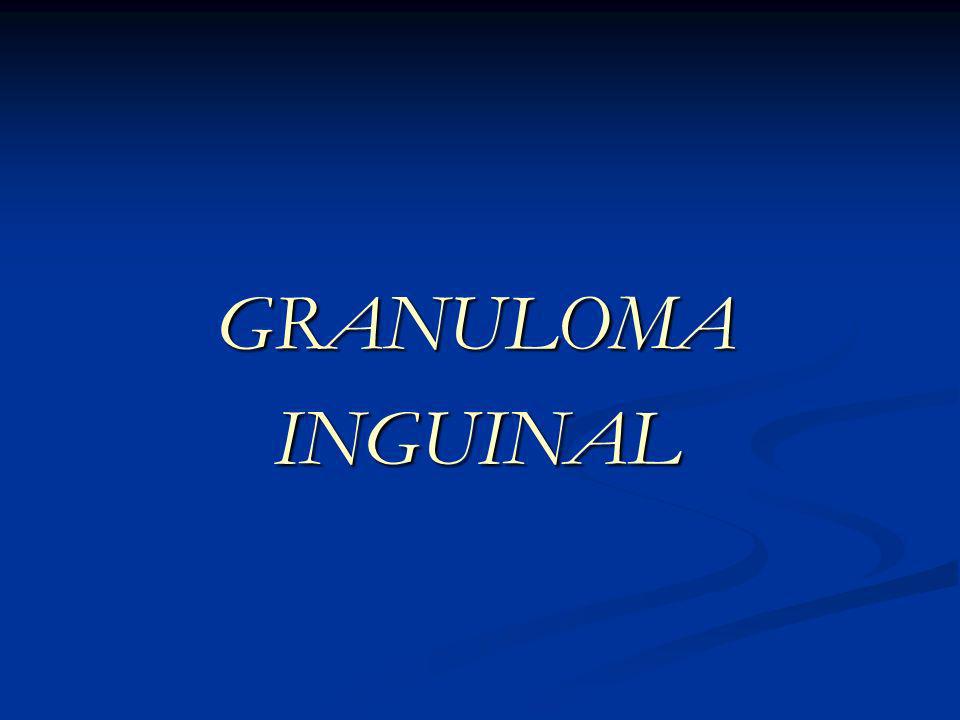The image features a gradient background transitioning from black at the top to a medium bright blue at the bottom. In the center, white, all-capitalized text reads "GRANULOMA INGUINAL." The background also includes a series of dark blue squiggly lines that start from the bottom right corner and curvily traverse towards the left, reminiscent of a winding road or pathway.